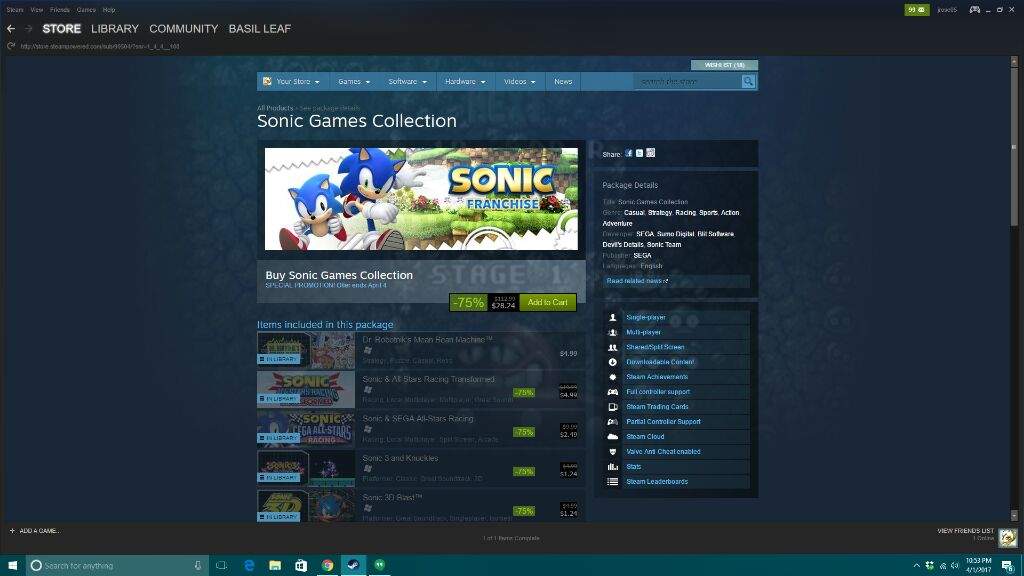This image depicts a classified section from a video game storefront interface. At the very top of the screen, a black banner displays the text "Store" in bold white letters. Next to it, in non-bold white letters, the banner features the options "Library," "Community," and "Basil Leaf," each spaced out evenly.

Directly below the black banner, the main interface has a dark blue background resembling a webpage or game screen. This area includes a lighter blue banner labeled "Your Store," followed by toggle options: "Games," "Software," "Hardware," "Videos," and "News," each accompanied by a caret symbol indicating they can be expanded.

Beneath this navigation bar, the white text reads "Sonic Games Collection," alongside two images of Sonic the Hedgehog accompanied by the inscription "Sonic Franchise." Following this, the caption "Buy Sonic Games Collection" appears in white, with a special promotion code offer ending on April 14th highlighted in light blue font. Below this, a green box displays "-75% Add to Cart."

Adjacent to the green discount box, there are additional options including "Share" and "Package Details," though these are not clearly readable in the image. The remainder of the screen seems to be filled with various other clickable options, though these elements are somewhat blurry.